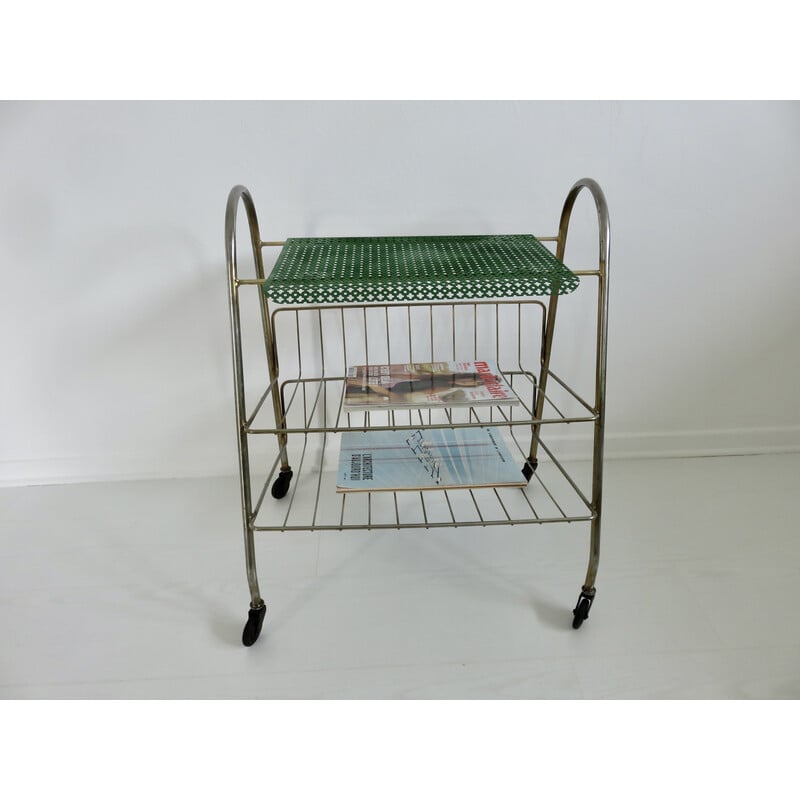This metal storage rack features an elegant design with two curved sides forming four legs, each equipped with a black wheel for easy mobility. The top of the rack is adorned with a green piece of fabric or plastic stretched across, adding a touch of color. The middle tier showcases a wire rack holding a magazine, utilizing the open structure to keep the item visible and accessible. Below, the bottom wire rack similarly supports a blue magazine or book. Both racks are designed with a back panel that rises slightly, ensuring that items remain securely in place, while the open wire construction provides a modern and airy aesthetic.